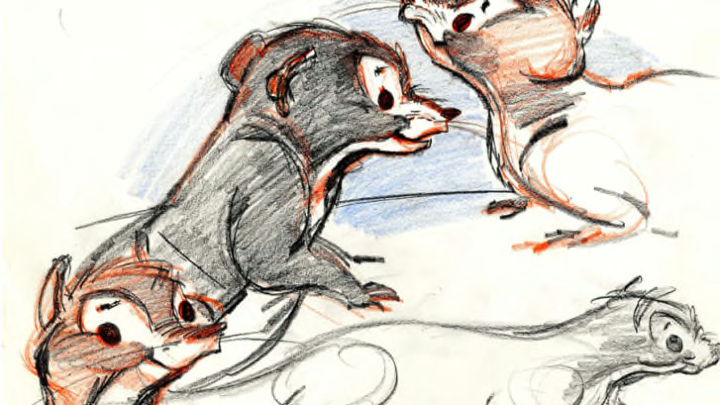The image displays a series of preliminary sketches, likely intended as the initial phase of an animation or cartoon. The drawing features four rodent-like animals, possibly mice or chipmunks, illustrated with varying degrees of detail and color. In the lower right corner, one of the rodents is sketched in black and white, with darker shading around the head, yet is otherwise uncolored. To the left of this figure, another rodent's head pops up, rendered with a mix of black, brown, and white. This one appears to be smiling and has a more defined, though still sketch-like, appearance. Above this head, another rodent is depicted with its full body visible, shaded predominantly in black with brown and white accents on its face. Finally, in the upper right corner, another rodent's body, mostly white with some brown and black around the head, is partially visible. The artwork appears to be created with colored pencils or similar medium, and despite its incomplete state, it hints at an engaging and lively set of characters.